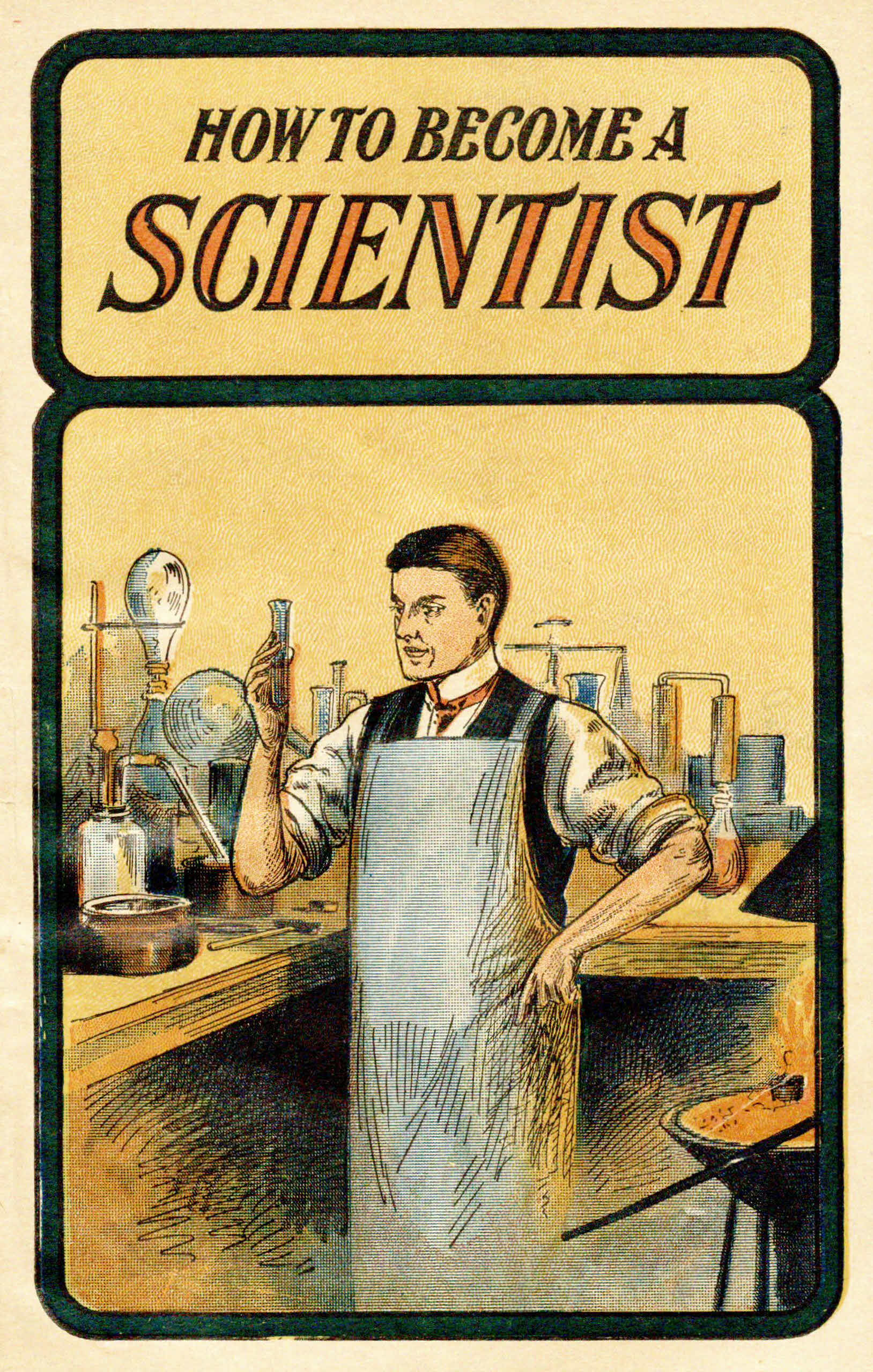The image appears to be an antique illustration, possibly from an old sign, card, or a book. The border of the image is a light beige-pink color, giving it a vintage aesthetic. The artwork is divided into two sections: the top section is a horizontal rectangle outlined in a dark forest green, while the bottom section is a larger vertical rectangle, outlined in the same dark forest green.

In the top section, the text "How to Become a Scientist" is prominently displayed, with the word "scientist" rendered in orange-red letters. The bottom section of the image features a detailed drawing of a Caucasian man, presumably a scientist, engaged in scientific work. He wears a vest, a long-sleeved white shirt possibly complemented by a tie, and an apron that appears to be gray or white.

The setting shows the man standing behind a light wooden countertop that wraps around a corner, laden with various scientific instruments. These include test tubes, clear bottles, hoses, and other laboratory equipment, indicating he is conducting experiments. To the right bottom, there is a scientific apparatus on black legs with a small controlled flame, possibly used for heating the test tubes or other materials. Additionally, there is a copper-colored bowl adjacent to the flame.

Overall, the illustration captures an intricate and historically-styled depiction of a scientist at work in his laboratory.